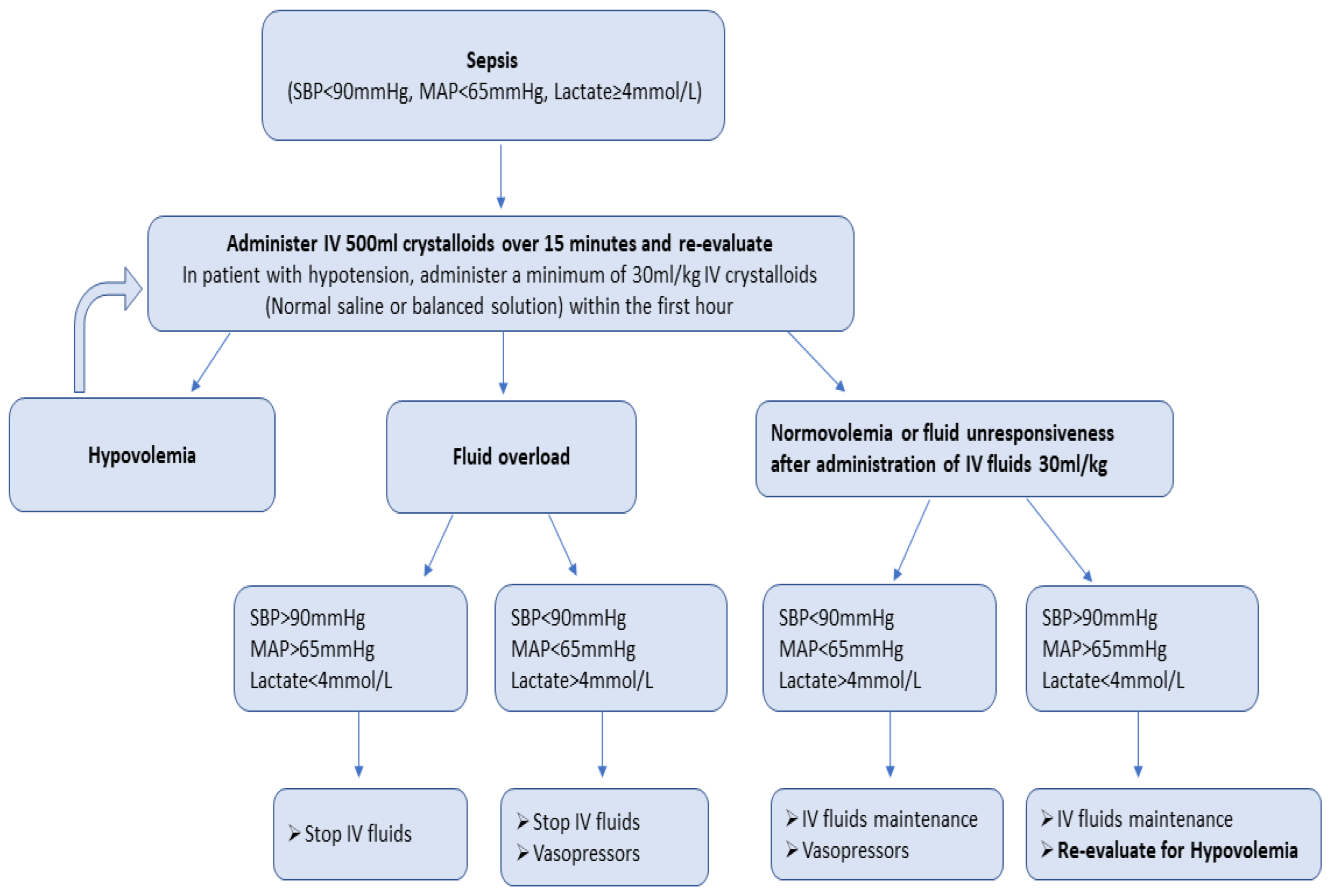The image is a detailed medical decision-making flow chart for managing sepsis, featuring multiple blue rectangles with rounded corners and dark blue borders. At the top, a bold black text box labeled "Sepsis" serves as the header. Below this, the chart advises to administer IV 500 milliliters of crystalloids over 15 minutes and then reevaluate the patient's condition. The subsequent decisions are based on the patient's fluid status: fluid overload, normovolemia, fluid unresponsiveness after IV fluids, or hypovolemia. 

For fluid overload, the chart indicates evaluations based on SPB (Systolic Blood Pressure) and MAP (Mean Arterial Pressure) levels, with thresholds set at SPB > 90 mmHg, MAP > 65 mmHg, and lactate levels < 4. If SPB is less than 90 mmHg, MAP is less than 65 mmHg, and lactate is greater than 4, fluid administration should be stopped, and vasopressors should be used.

Under normovolemia, similar evaluations of SPB and MAP are made. If SPB is less than 90 mmHg, MAP is less than 65 mmHg, and lactate is greater than 4, IV fluids maintenance and vasopressors are recommended. For SPB greater than 90 mmHg, MAP greater than 65 mmHg, and lactate less than 4, the chart suggests maintaining IV fluids and reevaluating for hypovolemia. Hypovolemia directs a return to administering IV fluids as needed.